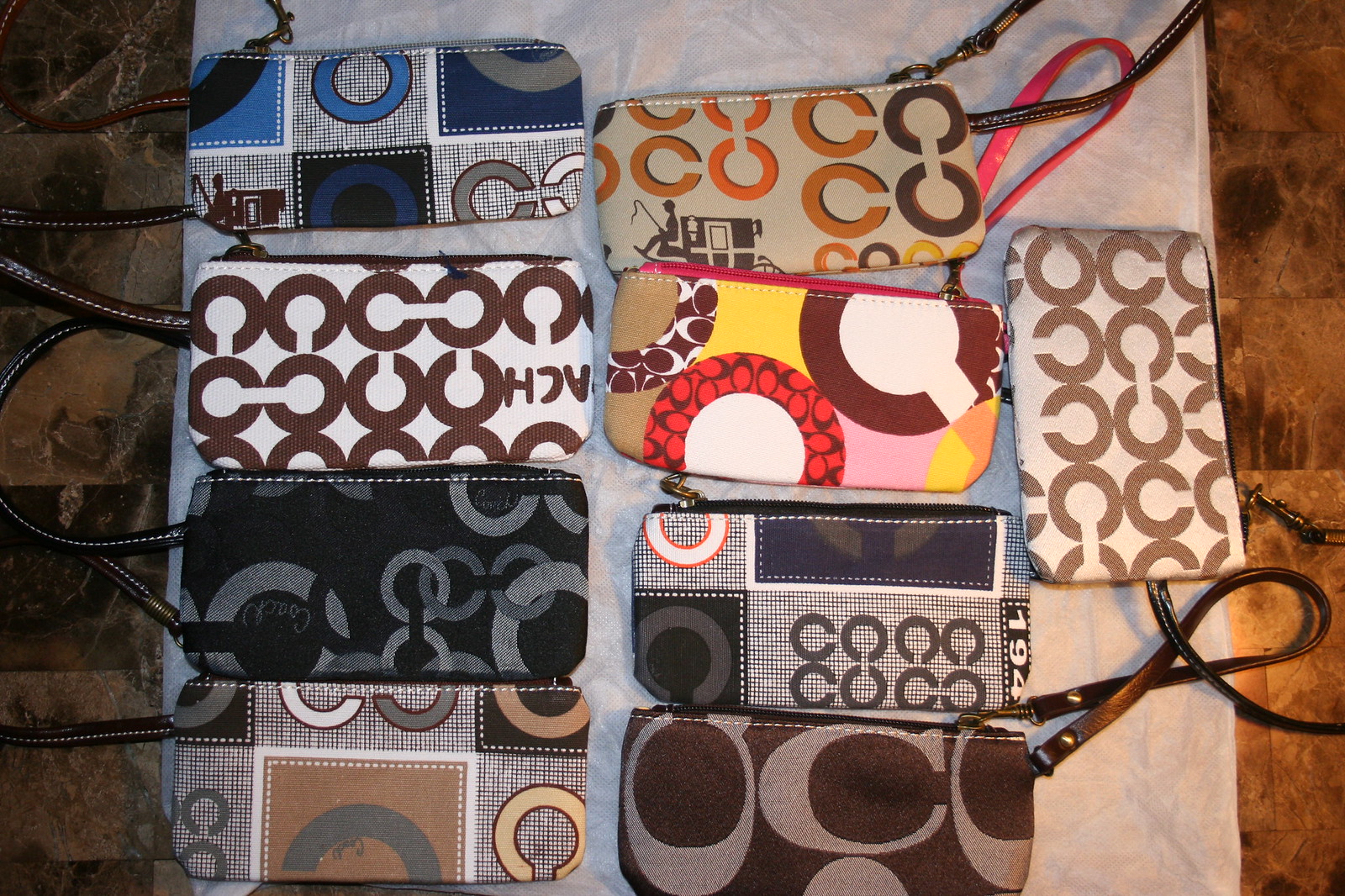In this photograph, an array of nine colorful wristlet bags, predominantly from the brand Coach, are meticulously arranged on a piece of light-colored, possibly gray, fabric that is set against a backdrop resembling grayish-brown marbled or imitation stone tiling. The wristlets are organized in a 2x4 grid with one sitting alone slightly off-grid, showcasing their uniform rectangular shapes with rounded edges. Each wristlet features a long, slim strap, some in black or brown leather-look material, and one with a distinctive pink strap. The bags are designed with various multicolored patterns, including cream, gray, blue, beige, brown, navy blue, red, pink, yellow, and white, all prominently adorned with the iconic Coach "C" insignia in varying sizes and styles. A few of the wristlets also explicitly display the "Coach" brand name, underscoring their designer origin. This image seems to be thoughtfully laid out, perhaps for display or sale purposes, capturing the elegance and diversity of the collection.